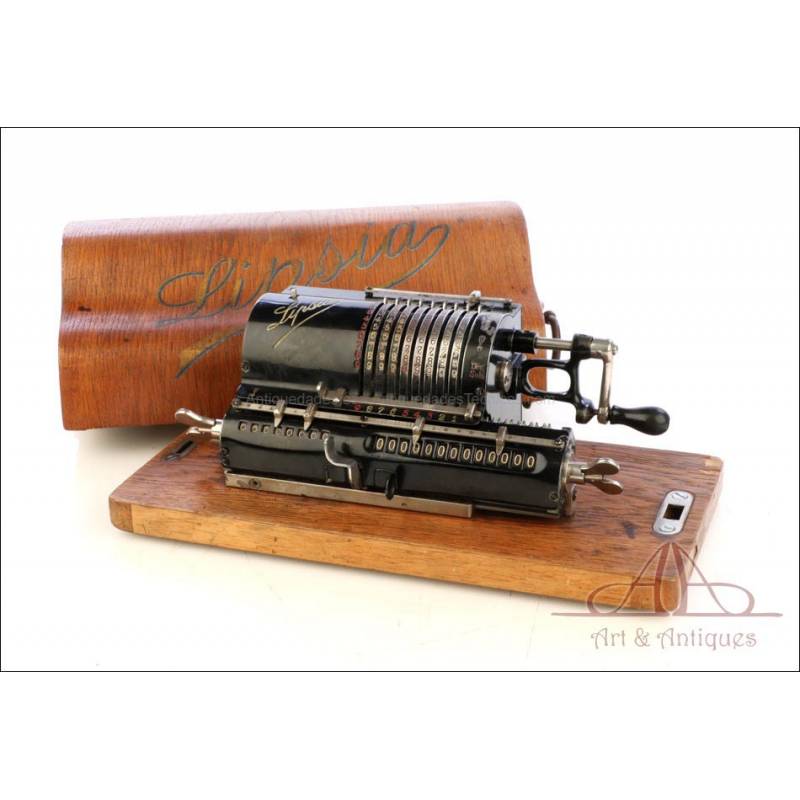This color photograph, presented in landscape orientation with a white background, captures an antique mechanical calculator known as a Lipsia. The machine is constructed predominantly of black metal and features a cylindrical top section with a squarish base beneath it. Attached to a shallow, dark brown wooden base with rounded corners and measuring about half an inch high, the calculator is equipped with a turn crank handle on the right side. The handle is chrome-colored with a black knob, and there are knobs on the side potentially used for tightening or adjustments.

The base shows distinctive silver elliptical bolt area on the right, while behind the calculator rests a wooden dome-shaped cover. The cover is adorned with a gold script logo reading "LIPSIA," complete with a black shadow and a decorative swash underneath. The calculator itself includes rows of numbers with sliding adjustments for selecting and imprinting numbers, indicated by squared white zeros.

Additionally, the machine exhibits characteristics akin to a music box, with some features resembling coins or musical elements visible. The overall aesthetic and design elements suggest a finely crafted, antique piece. In the bottom right corner of the photograph, there is a logo featuring two A's back-to-back, and beneath it, the text "Art and Antiques" in vintage light brown typography. This detailed setup enhances the perception of the calculator as both a functional device and a valuable antique art piece.